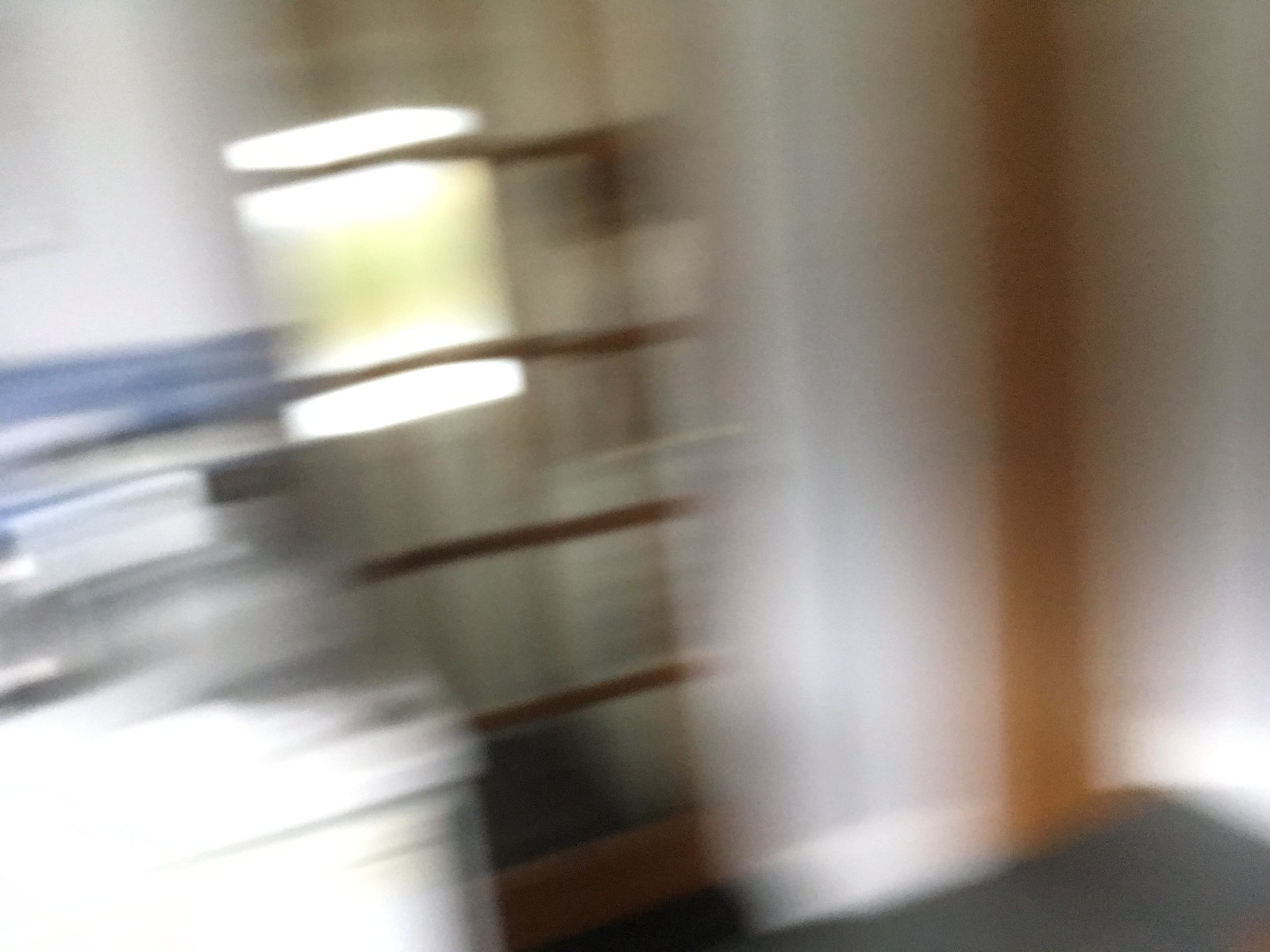This image, though very blurry, captures a kitchen scene with several identifiable elements. In the foreground, the floor appears black. At the center of the frame, wooden structures extend vertically and horizontally. On the right side of the image, there is a prominent white wall. To the left side, some white features are visible, and further to the far left, a stovetop with small silver knobs can be discerned. The base of the stove has a white trim. Above the stove, a strip of blue tile runs horizontally.

At the very top of the image, the wall is white, reflecting light. A partially open window creates a reflection, diffusing white light at the top and bottom, while green hues fill the middle of the window. Brown strips frame the door, and there are glass squares on the windows. Despite the blurriness, these elements collectively form a rustic, slightly chaotic kitchen atmosphere.